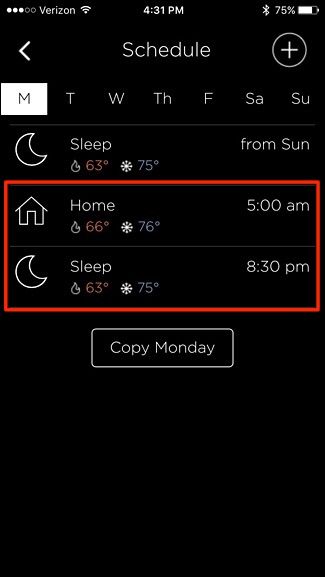This is a detailed descriptive caption for an image captured from a mobile device screen:

The screenshot appears to be from a cell phone or tablet. In the top-left corner, there are five white circles indicating signal strength; three circles are filled-in, signifying connectivity, while two circles are outlined but not filled, indicating lower signal strength. To their right, there is a white text displaying "Verizon" followed by a full Wi-Fi signal icon. Centered at the top of the screen, the time reads 4:31 PM. To the right of the time, the Bluetooth icon is visible, and the battery percentage shows 75%.

Just below the status bar, there is a navigation arrow pointing left. The text "Schedule" is prominently displayed in white. To the right of "Schedule," there is a white circle with a plus sign inside it. Below this bar, the days of the week are listed in abbreviated form: "M" for Monday, "T" for Tuesday, "W" for Wednesday, "TH" for Thursday, "F" for Friday, "SA" for Saturday, and "SU" for Sunday. Monday is highlighted within a white rectangle, indicating it is currently selected.

Below the weekdays, there are various indicators. A crescent moon icon is labeled "Sleep." Next to it is a flame icon with the text "63%" in red, likely representing a certain metric or a usage statistic. Adjacent to this is another icon resembling a snowflake or possibly raindrops, showing "75%," and the text "from Sunday."

Further down, in a section marked with a red outline, there is another schedule indicator showing "Home" next to a house icon. This section also lists percentage values: "66%" next to a flame icon and "76%" next to a snowflake. The time listed here is 5:00 AM, followed again by a crescent moon icon labeled "Sleep," and repeated metric values: the flame icon marked "63%" and the snowflake "75%," followed by the time 8:30 PM.

At the very bottom of the screen, inside a white-outlined box, the text reads "Copy Monday."